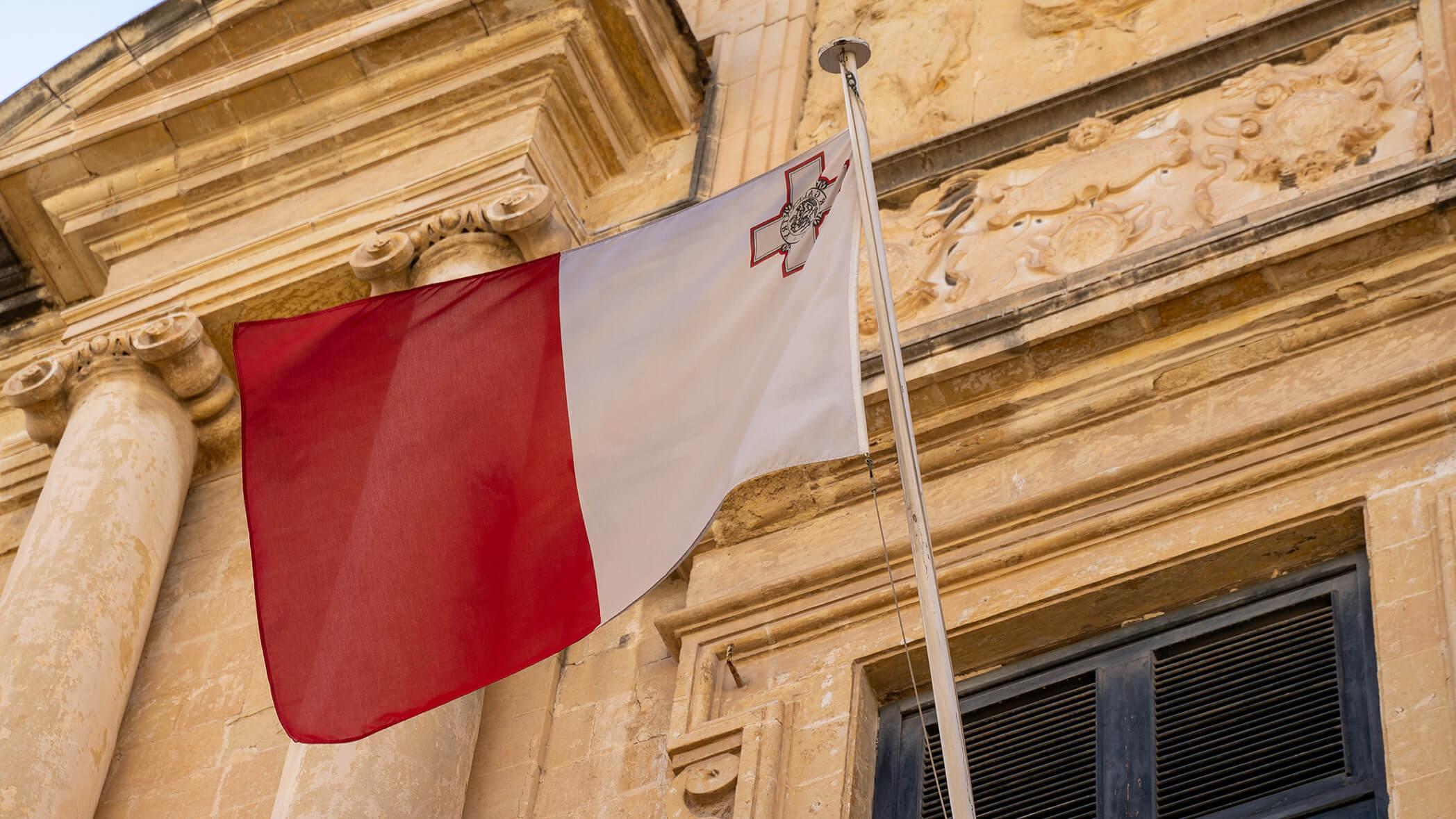This is a photograph of an old, vintage stone building, evocative of European architecture. The building's facade, captured from a ground view looking upwards, showcases intricate detailing on the columns, including elaborate carvings and stylized "curly cues" at the top. The stone appears to be a brownish hue, similar to marble. Central to the image is a silver flagpole extending from the building, displaying a flag that is half red and half white. On the white section of the flag, there's a cross outlined in red, with the cross itself appearing to be a cream or off-gray color. Additionally, a black shutter can be seen covering a window in the lower right portion of the image. The scene is devoid of people, focusing entirely on the architectural and historical elements of the building and the prominently featured flag.